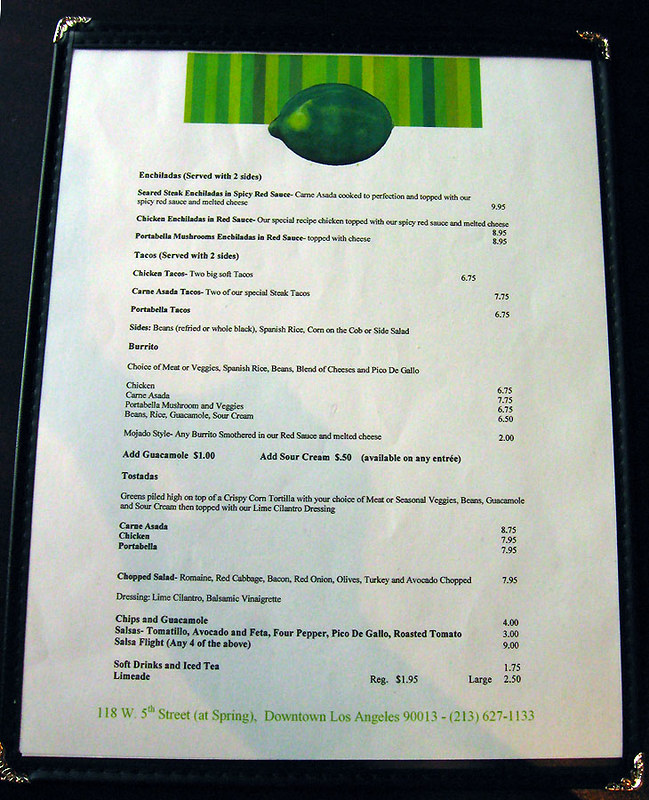**Descriptive Caption:**

The image displays a menu from a Mexican restaurant located in downtown Los Angeles at "118 West 5th Street at Spring, Downtown Los Angeles, CA 90013". The contact phone number for the restaurant starts with the 213 area code. The menu, printed on a single laminated sheet with a white background and a green stripe near the top, features a variety of Mexican dishes, including enchiladas, burritos, tacos, and tostadas. Specific items and prices listed include a carne asada tostada for $8.75, chips and guacamole for $4, and a chopped salad for $7.95. Additionally, limeade is offered at $1.95 for a regular size and $2.50 for a large.